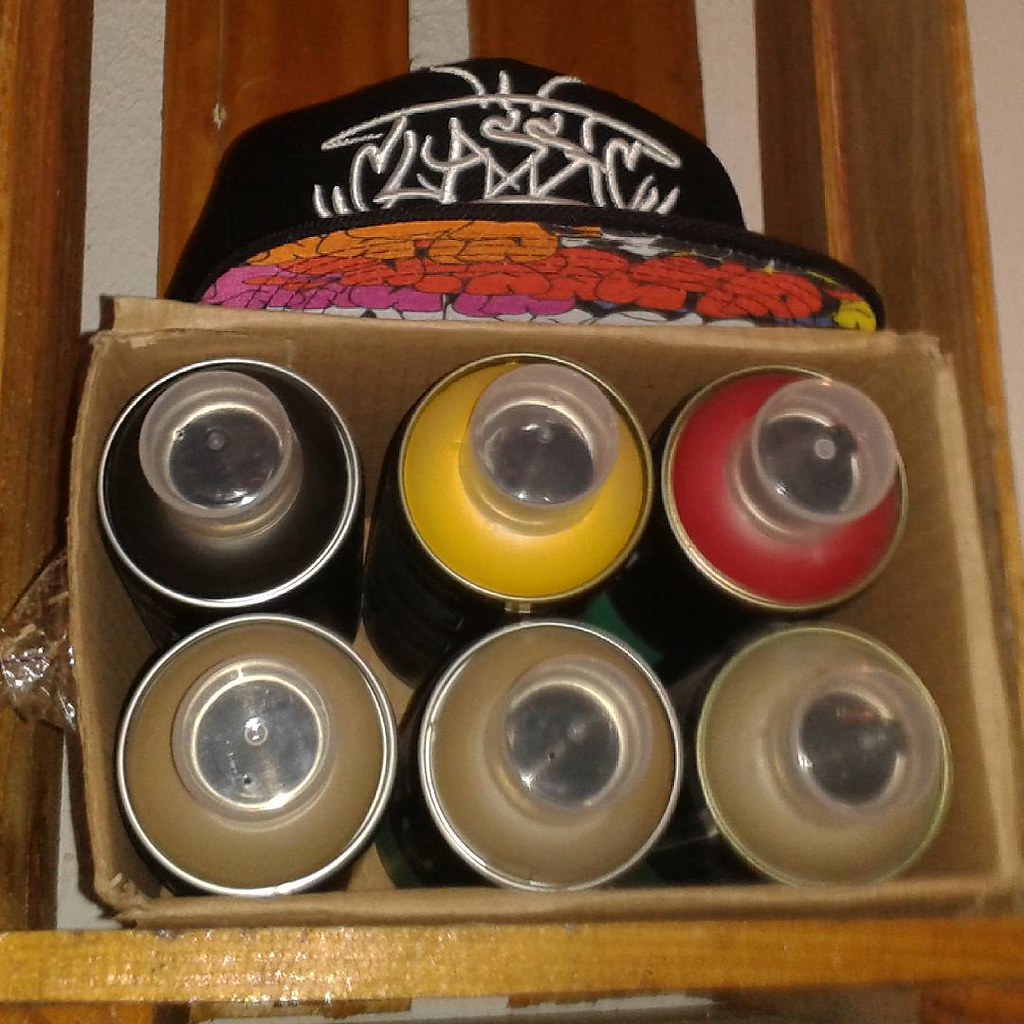This photograph captures a scene featuring a cardboard box positioned on its side on a wooden shelf. Inside the box are six cylindrical cans, arranged in two rows of three. From our vantage point, we see their tops clearly: the top row comprises cans with black, yellow, and red tops, while the bottom row consists of cans with tan tops. Each can has a silver-rimmed lid and a clear plastic center, suggesting they might contain spray paint or some other substance. Perched atop the box is a black baseball cap adorned with unreadable white text on the front and vibrant graffiti-style artwork in orange, red, pink, and yellow on the underside of the brim. The background includes wooden paneling and white stucco walls, enhancing the rustic ambiance of the scene. The wooden shelf has a lighter brown base with cherry-toned sides, adding to the warm, contrasted texture.